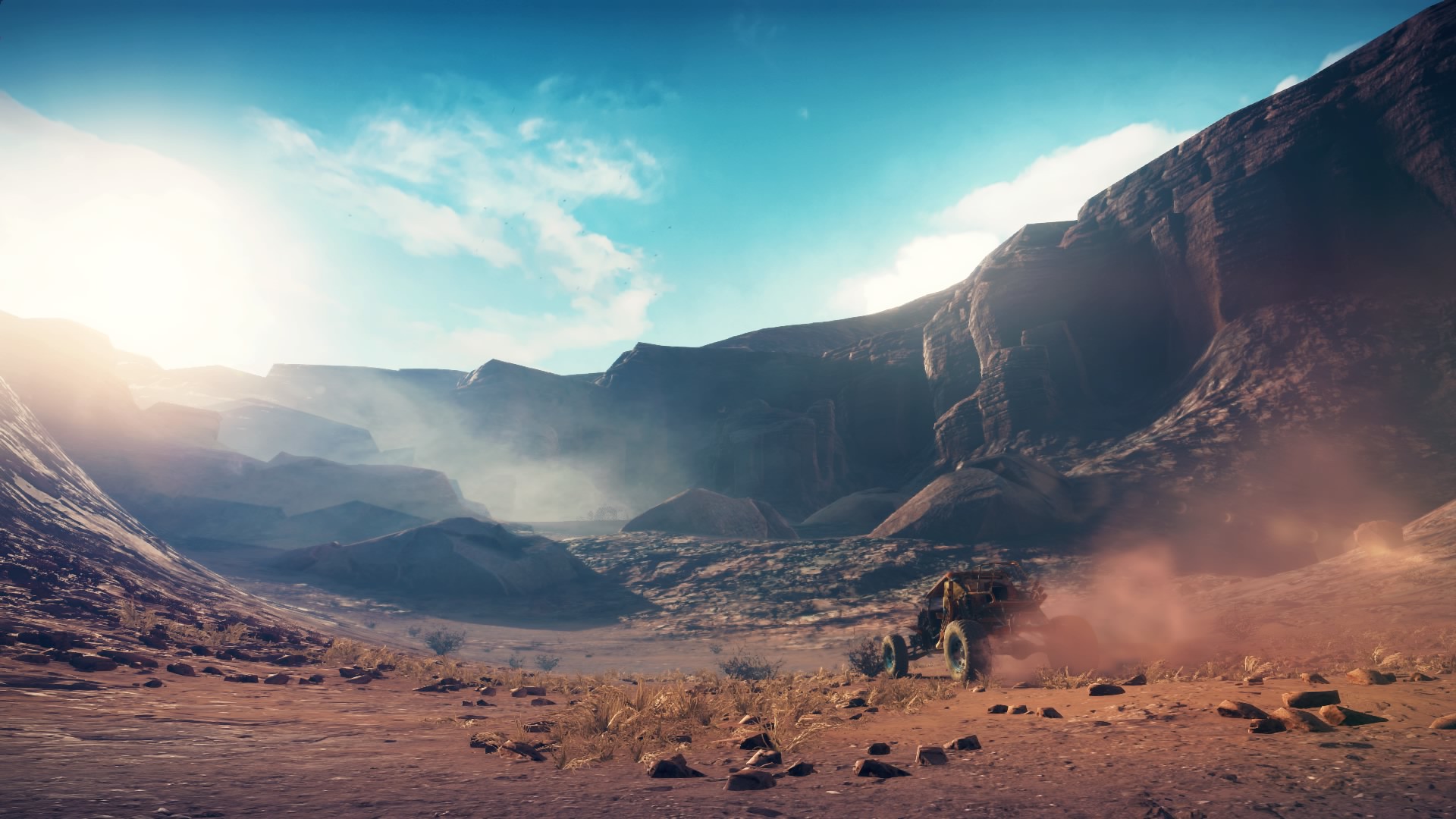A striking photograph captures a large, four-wheeled vehicle, predominantly yellow with contrasting black wheels, as it traverses a rugged desert landscape. The vehicle appears somewhat distant, making its exact model hard to discern. The foreground is scattered with tan-colored sandy dirt and sporadic rocks. The background features an array of rock formations of varying heights, in hues of tan and darker brown. Dust and sand are visibly kicked up by the vehicle’s movement, adding to the dynamic feel of the scene. Above, a brilliant blue sky dotted with fluffy white clouds stretches across the horizon. Small patches of desert grass dot the landscape, adding a touch of greenery to the arid environment.